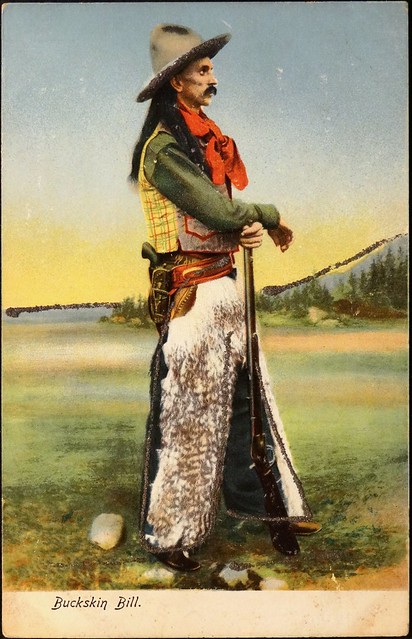This image depicts Buckskin Bill, prominently labeled at the bottom in black print. The scene appears to be an old-timey, early 20th-century colored drawing or painting, possibly reminiscent of a vintage postcard in a vertical format. Buckskin Bill stands in an expansive, flat prairie landscape with grass, trees, and rocks, with a hill or small mountain featuring whitish coloration in the distance. The sky takes on a golden tone, suggesting it might be dusk.

Buckskin Bill is dressed in traditional cowboy attire: a flat gray cowboy hat, a green buttoned shirt, a yellow and gray vest, and white cowskin chaps over his pants. Around his neck is a red kerchief. He has a holster with a revolver on his right hip and is holding a shotgun, its barrel resting on the ground, with both hands. Bill appears to be posing and is looking off to the right, showing his profile, which is characterized by long black hair and a handlebar mustache.